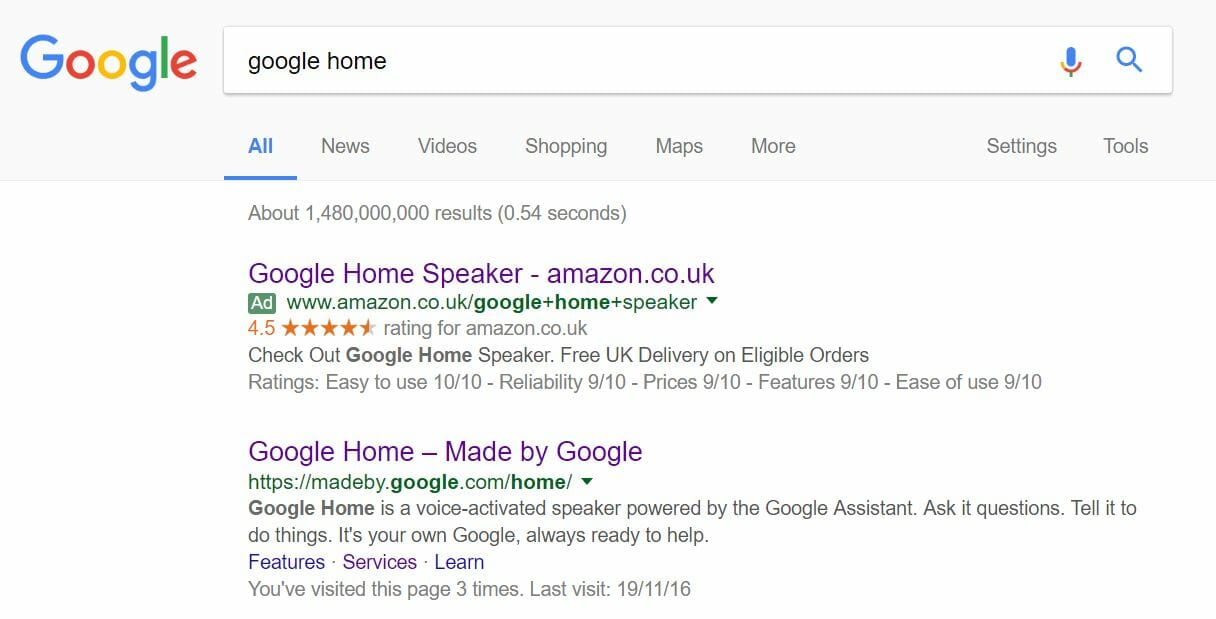Here is a refined and detailed caption for the image:

---

A screenshot of a Google search results page is displayed. At the upper left corner, the iconic Google logo is prominently featured in its multicolored lettering. To the right of the logo, the search bar contains the search term "Google Home," accompanied by a microphone icon and a magnifying glass icon on its right side. 

Beneath the search bar lies a row of search categories listed from left to right: "All," "News," "Videos," "Shopping," "More," followed by "Settings" and "Tools" on the far right. 

The search results are focused on "Google Home," with the top results showcasing links such as "Google Home Speakers | Amazon.co.uk," which highlights free UK delivery on eligible orders, and "Google Home - Made by Google," describing it as a voice-activated speaker powered by the Google Assistant. 

The results emphasize the convenience and functionality of Google Home products, catering to users in the UK market.